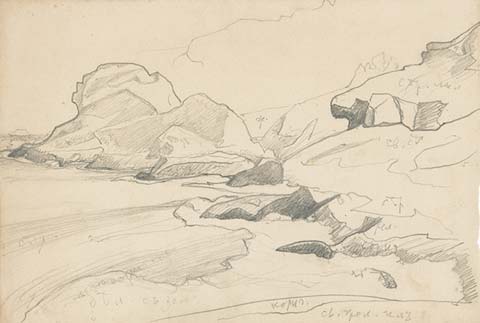This black and white drawing, rendered in what appears to be gray pencil or possibly charcoal, depicts a serene landscape dominated by rock formations. The majority of the image consists of a cream-colored background, providing a subtle contrast to the grayish sketches. Throughout the piece, different rock formations are carefully illustrated, some shaded to suggest depth and texture, while others remain clear and unshaded. At the top of the drawing, softly outlined clouds drift across the sky, adding to the atmospheric feel of the scene. The terrain of the land is meticulously outlined, with what could be a hillside or stylized beach to the left and a river or winding pathway moving through the scene. Scattered among the rocks, bits of grass seem to be growing next to them. There appears to be a faint, almost lightning-like crack in the sky, which might actually be distant mountains. Furthermore, the drawing includes some discolored areas, likely from sketch doodles, and there are indistinct writings toward the bottom right. The name of the artist can be faintly seen in the bottom right corner, though it is quite difficult to read due to its light application.